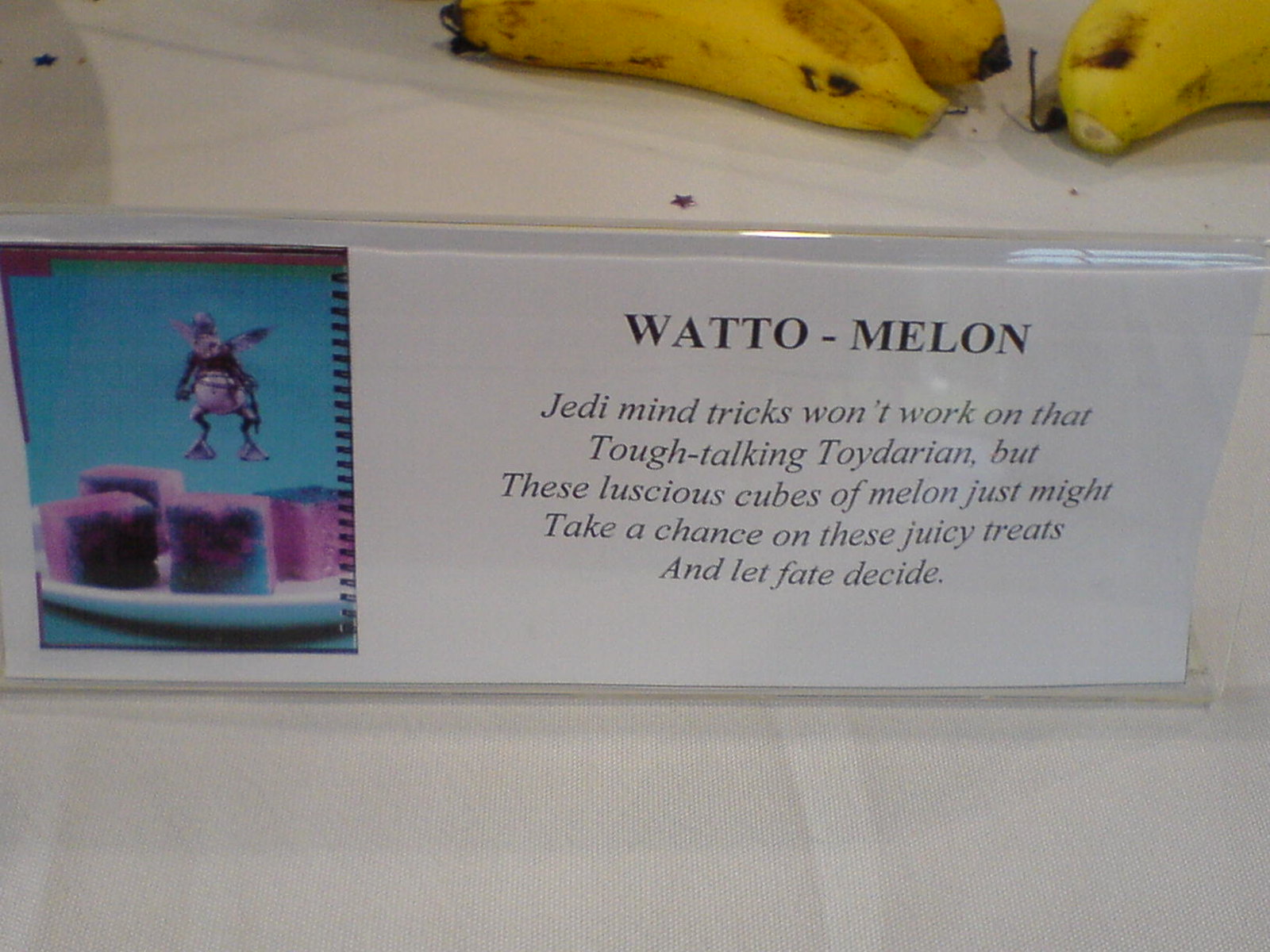The image showcases a detailed indoor scene set on a table draped with a white tablecloth. Prominently featured is a small glass sign board. On the left side of this sign, there's a somewhat blurry picture depicting cubes of melon with what appears to be an insect flying above them, against a blue background. The right side of the sign displays black text on a white paper that reads "Waddle Melon. Jedi Mind Tricks won't work on that tough talking Toydarian, but these luscious cubes of melon just might. Take a chance on these juicy treats and let fate decide." Additionally, the top right of the image features three small bananas.